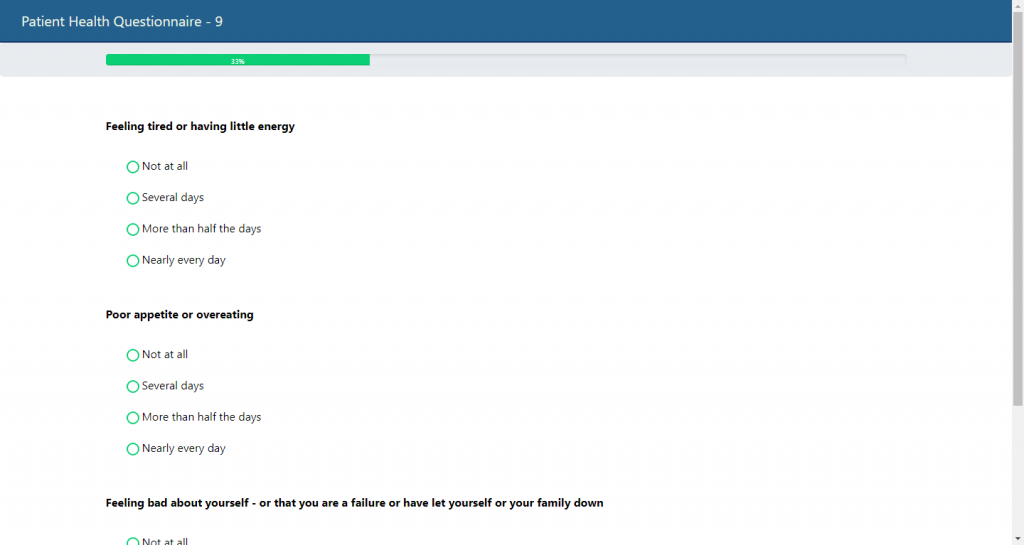This image is a detailed screenshot of page 9 from an online Patient Health Questionnaire. At the top of the screenshot, there's a dark blue horizontal bar with the title "Patient Health Questionnaire 9" displayed in lighter, almost white, capital letters. Below this title, there's a progress bar indicating the user's completion status; approximately 35% filled, colored in a bright light green, although the exact percentage is hard to discern due to the small screen size.

The main body of the screen captures the actual questionnaire, showcasing a series of questions and multiple-choice answers. The visible questions include:

1. "Feeling tired or having little energy?" with answer options:
   - Not at all
   - Several days
   - More than half the days
   - Nearly every day

2. "Poor appetite or overeating?" with similar response choices:
   - Not at all
   - Several days
   - More than half the days
   - Nearly every day

3. "Feeling bad about yourself or that you are a failure or have let yourself or your family down?" The screen shows only part of the "Not at all" option, with the rest cut off by the bottom of the display.

This screen forms part of a larger questionnaire aimed at assessing the patient's health and well-being through progressively detailed inquiries.